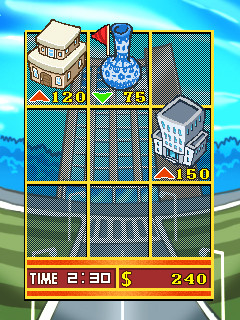This image appears to be a screenshot from a game, presented in a cartoon-style artwork. Central to the image is a 3x3 grid, containing various objects and symbols. In the top row, the first square on the left features a two-story tan house with a white roof. Below the house, a red arrow pointing upward reads "120." Adjacent to this, in the second square of the top row, is a blue vase adorned with white decorations. To the left of the vase is a red flag, and beneath it, a green arrow pointing downward with the number "75." The second row's third square contains a white office building resembling a hospital, with a red arrow pointing upward below it that lists "150." Below the grid, there is an inscription that reads "time 230, s 240."